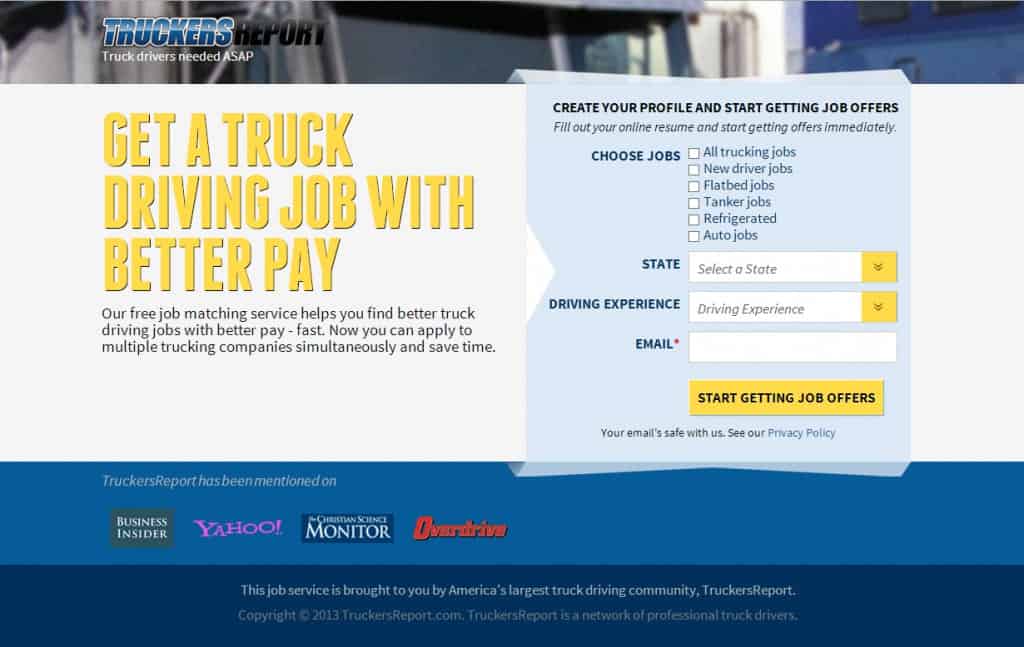This image is a screenshot of an opt-in form specifically designed for truck drivers seeking employment. The form prominently features the headline "Trucker’s Report: Truck Drivers Needed ASAP." Below this, a white section with yellow text urges drivers to "Get a truck driving job with better pay."

The form includes a detailed paragraph about job opportunities and is visually segmented into several color sections: a dark blue area and a light blue area. Below these sections, it states that job services are brought to you by America's largest truck companies, and mentions notable collaborators such as Business Insider, Yahoo, and Overdrive. The "Trucker’s Report" is also referenced.

Users are prompted to create their profile to begin receiving job offers. The form allows drivers to choose from various job categories, including "All Trucking," "New Trucking," "Flatbed Jobs," "Tanker Jobs," "Refrigerated Jobs," and "Auto Jobs." It also includes fields for selecting the state and specifying driving experience, followed by an email address input. A note assures users that their email is safe.

Additionally, the names of collaborating companies are highlighted in distinct colors: "Overdrive" is written in red, "Yahoo" in purple, and "Business Insider" appears within a gray square with white lettering.